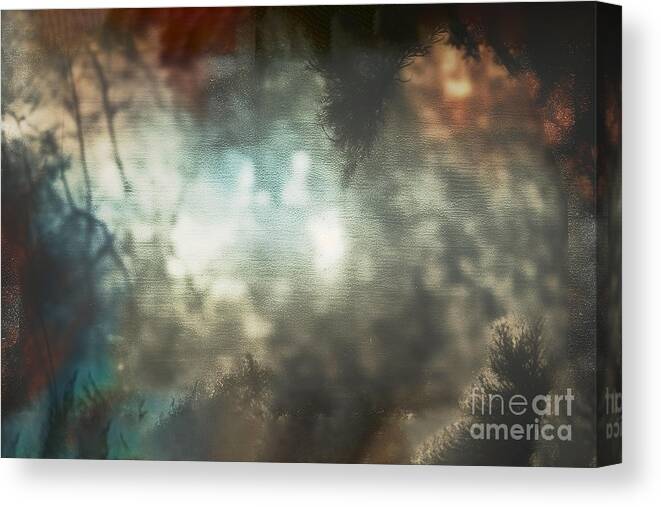This image features a wraparound canvas displaying a photograph, possibly with filters, capturing an enigmatic, intentionally blurred woodland scene for artistic effect. The image, titled "Fine Art America" as noted in the bottom right corner and mirrored along the side, presents a serene, almost dreamlike quality. Apparent is the essence of trees—both broadleaf and evergreen—creating a natural frame around the image. These trees, with their indistinct forms and scattered branches, evoke the sensation of lying in a forest glen, looking up through a hazy sky bathed in soft, diffuse light, suggesting either dawn or dusk.

The canvas exhibits a range of colors: dark greens, peach, and light blue, with tinges of red, yellow, and orange, giving a sense of seasonal transition—either late fall or early spring. The texture suggests a combination of photographic and painterly elements, with the foliage and fog merging seamlessly into the background, where patches of sky filter through the branchwork. Detailed features like the pine cone perched on the bottom right branch add to the forest ambiance. The scene, dominated by soft shades and a peaceful halo of light in its center, conveys tranquility and a meditative escape into nature’s quiet embrace.